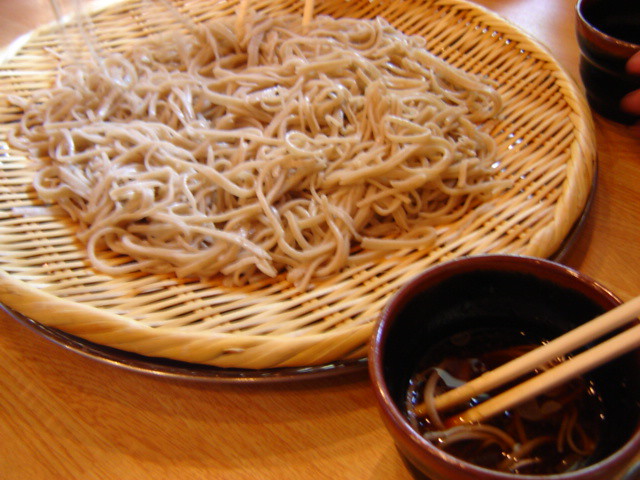The photograph captures an Asian-style dining setting featuring a traditional bamboo or straw mat acting as a communal plate for noodles. The intertwined strands of the mat create a slightly diagonal pattern, enhancing its rustic charm. Mounded on this woven mat are plain, light tan noodles that appear to be either fried or dried. Positioned around this central mat are various dining elements: in the bottom right corner, there's a small brown ceramic bowl filled with a dark sauce, presumably soy or a dipping sauce, with chopsticks poised to dip noodles into it. Another pair of chopsticks rests atop the noodles on the mat. Additionally, in the top right corner, there's a drinking cup with distinctive orange buttons on its edges, matching the small bowl's color. All these items are arranged on a light brown wooden table, indicative of a shared dining experience, possibly in a restaurant setting, where diners collectively partake from the central platter.